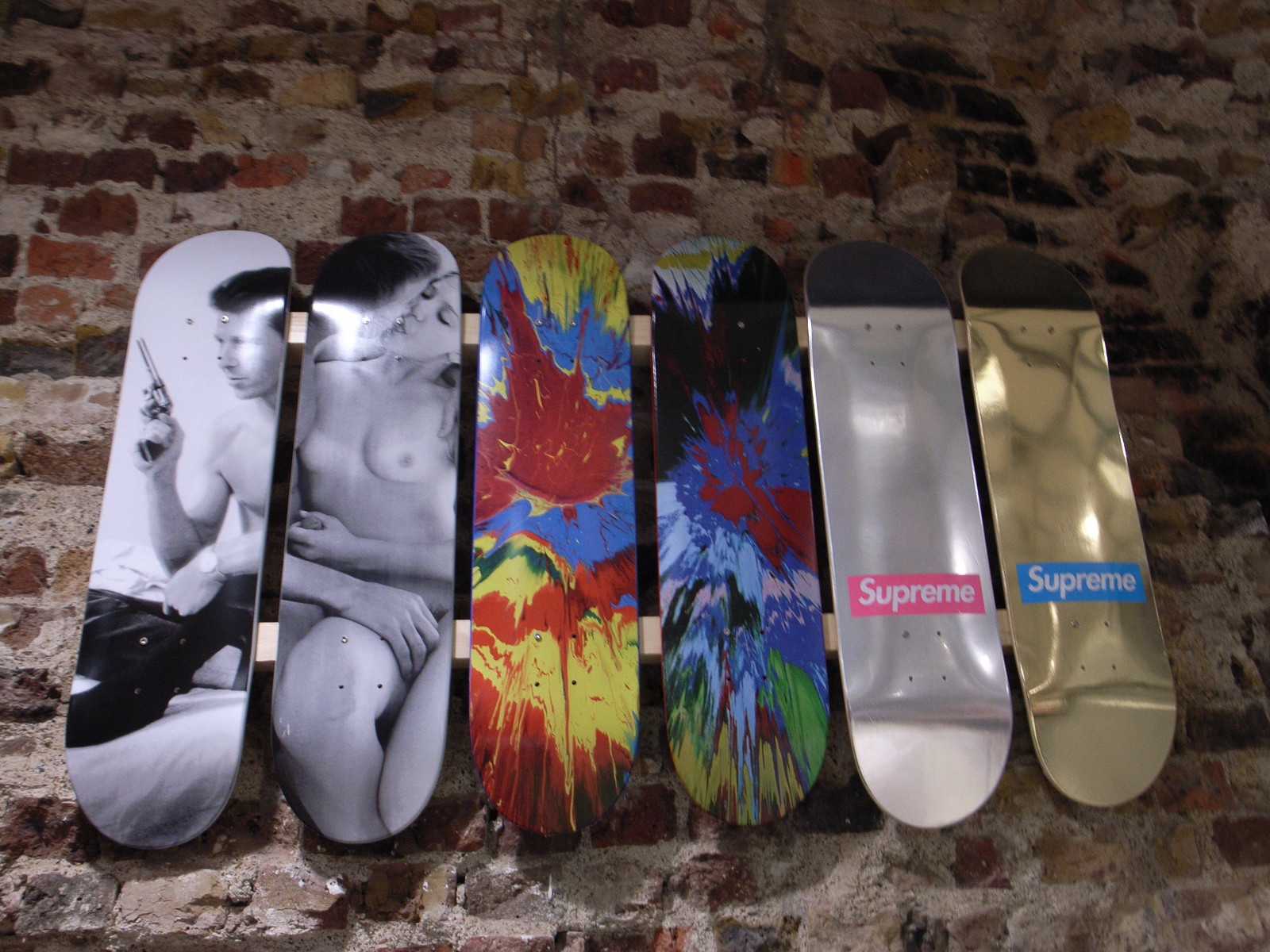The image showcases a display of six skateboard decks mounted against a distressed red brick wall, which provides a rich, textured background. These skateboards are arranged in a row and attached to two wooden supports. The first deck on the left features a black-and-white photograph of a shirtless man wearing darker pants, who holds a pistol in his right hand and a wristwatch on his left. The second deck displays another black-and-white image of a couple where the woman, who is naked, and the man are engaged in a passionate kiss, with the man's hand between her legs. The third and fourth decks exhibit a vibrant paint splatter or tie-dye effect in a myriad of colors, including reds, blues, yellows, greens, pinks, and blacks. The fifth deck is entirely silver with a black top and has a prominent Supreme box logo in white lettering on a pink background. The sixth and final deck is gold with a black top, and it also features a Supreme box logo, this time in white lettering on a blue background. The entire arrangement rests on a brick surface that complements the rustic look of the brick wall behind.